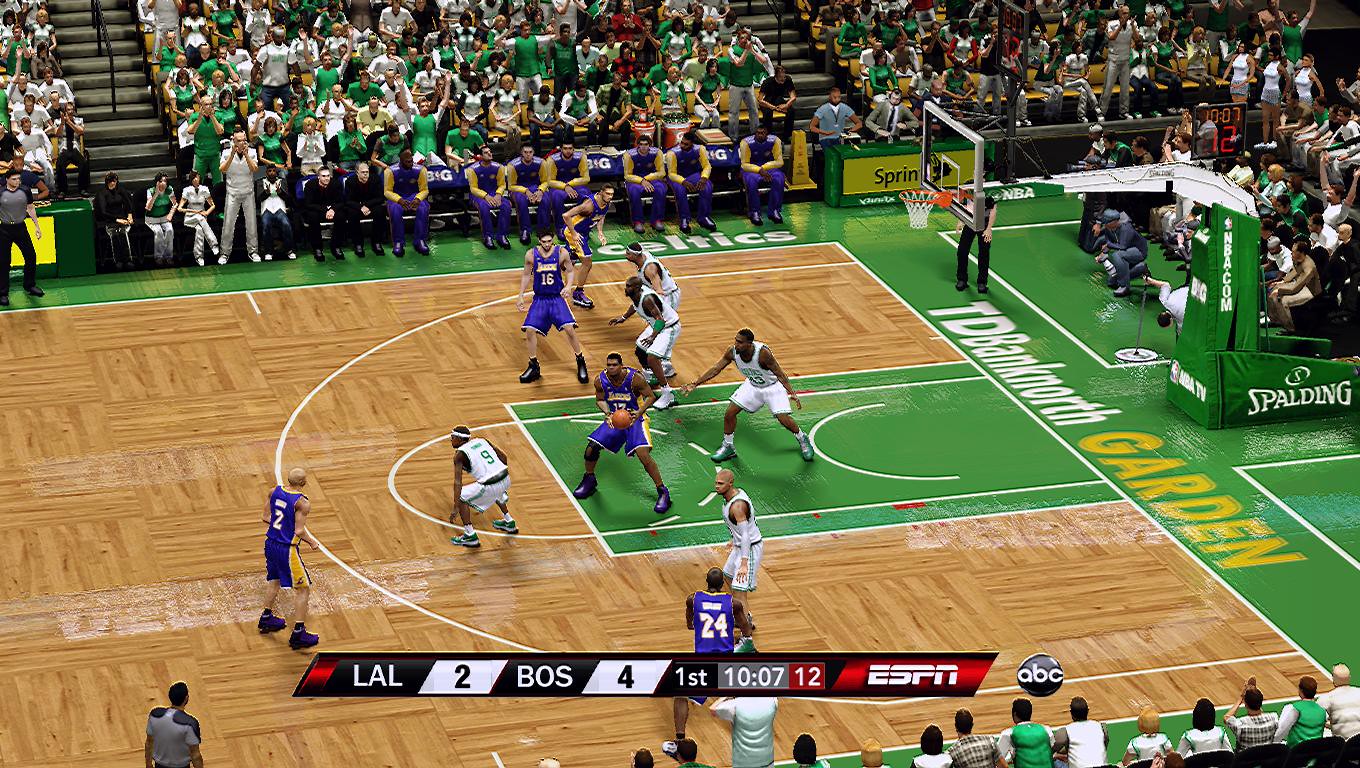A highly detailed and ultra-realistic still image from a basketball video game, showcasing half of the beautifully rendered wooden basketball court with a green-painted border. The court is identified as TD Banknorth Garden, prominently displayed along the side. The scene captures the tense moment of gameplay, featuring players from two iconic teams: the Los Angeles Lakers, dressed in their signature purple uniforms, and another team in crisp white jerseys. The scoreboard at the bottom reveals an early lead, with the Lakers (LAL) trailing the opposing team (presumably the Boston Celtics, BOS) by 2 points to 4, in the first quarter with 10 minutes and 7 seconds remaining. The game's broadcast is indicated by the ESPN and ABC logos.